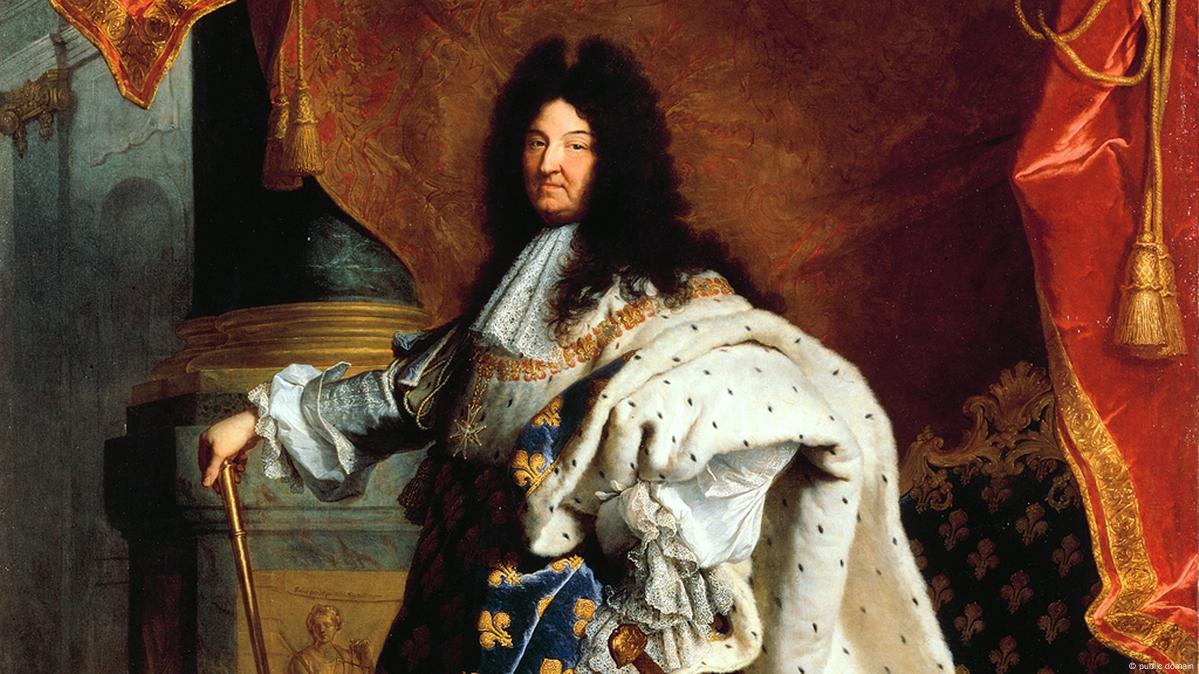This detailed full-color painting, a famous depiction from the 1700s, illustrates a French king, likely Louis XVI. The horizontally rectangular image, devoid of a specific background, features a white trademark at the lower right corner labeled 'Public Domain'. The painting centers an older Caucasian man with a full, curly black wig cascading over his shoulders and back. He exudes an air of wealth, conveyed through his attire: a thick, luxurious white and blue robe adorned with yellow club-like motifs, and a heavy, dark blue robe with ornate orange flower patterns. The king stands in a poised yet somewhat bored demeanor, his facial expression flat, and his bulky frame emphasizing his grandeur and opulence. His right hand is outstretched, gripping a gold walking stick, symbolizing authority. The scene is enriched with elaborate yellow and red curtains, accentuating the regal setting. The painting is a testament to the king's stature and the elaborate style of his time.